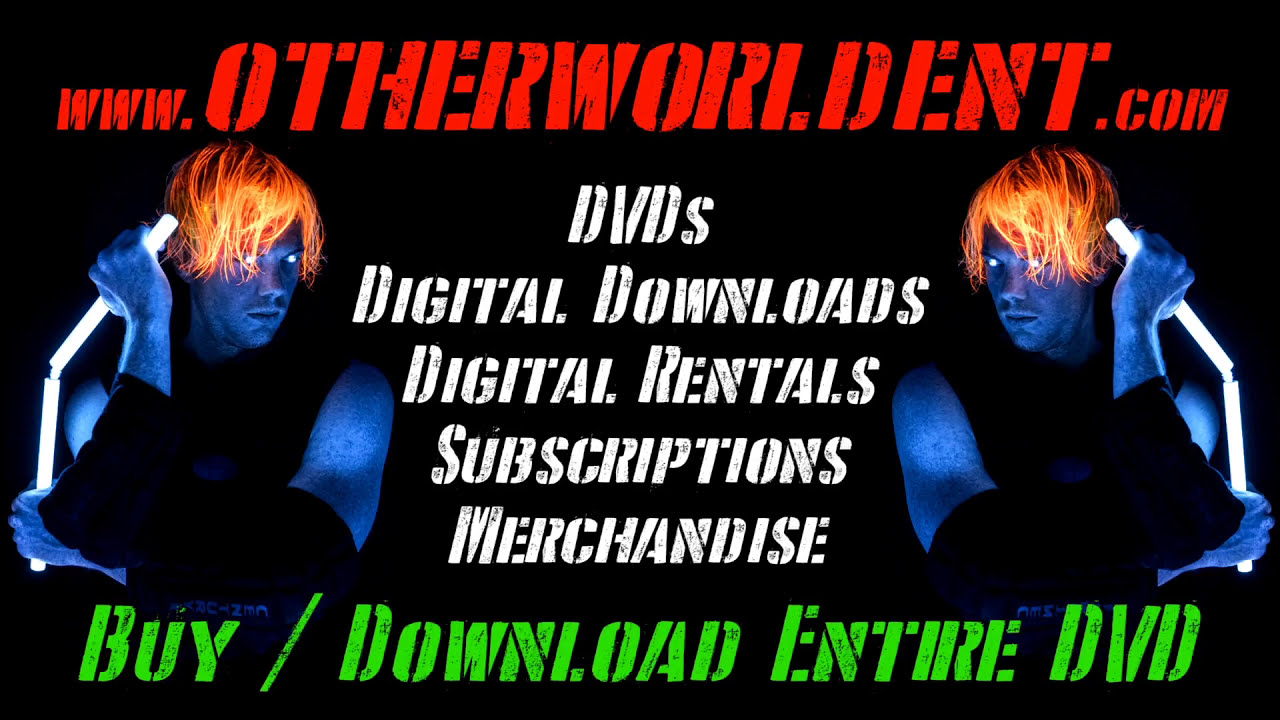The advertisement features a striking image highlighted by its dark backdrop with vividly colored elements. At the very top, in bold red text, it reads: "www.otherworlddent.com". Dominating the sides of the ad are mirror images of the same man, likely duplicated digitally. He has fiery, medium-length orange hair and piercing white, glowing eyes which give him an otherworldly appearance, akin to a video game character. His skin glows a bright, dark blue, possibly enhanced by blacklight effects. He wears a shoulderless black shirt and black elbow pads, holding glowing nunchucks in a martial arts stance with his right arm raised beside him and his left arm crossed over his chest. The centerpiece of the ad, positioned between the mirrored images of the man, lists the offerings in white text: "DVDs" on the first line, "digital downloads" on the second, "digital rentals" on the third, "subscriptions" on the fourth, and "merchandise" on the fifth. Below this, in green text, the message "buy/download entire DVD" runs horizontally, emphasizing the call to action. The overall aesthetic suggests an advertisement for a website offering action-packed entertainment products, including physical and digital media.